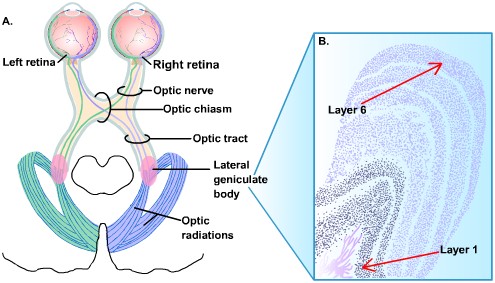This infographic features two labeled diagrams illustrating the visual pathway in the brain. The left side, designated as Figure A, starts with two peach-colored circles at the top representing the left and right retinas. Beneath these circles, a series of connected structures are depicted: the optic nerves originating from each retina, converging at the optic chiasm, and then splitting into the optic tracts. Further down, these tracts lead to the lateral geniculate body and continue as optic radiations. Each part is clearly labeled with black font, guided by small black bars.

On the right side of the infographic, labeled as Figure B, there's a large blue rectangle featuring light purple curved swirls, visually similar to a thumbprint. Two red arrows are present within this rectangle, pointing to specific layers labeled 'Layer 6' at the top and 'Layer 1' at the bottom. This section provides a detailed visual of the different layers within the lateral geniculate body.